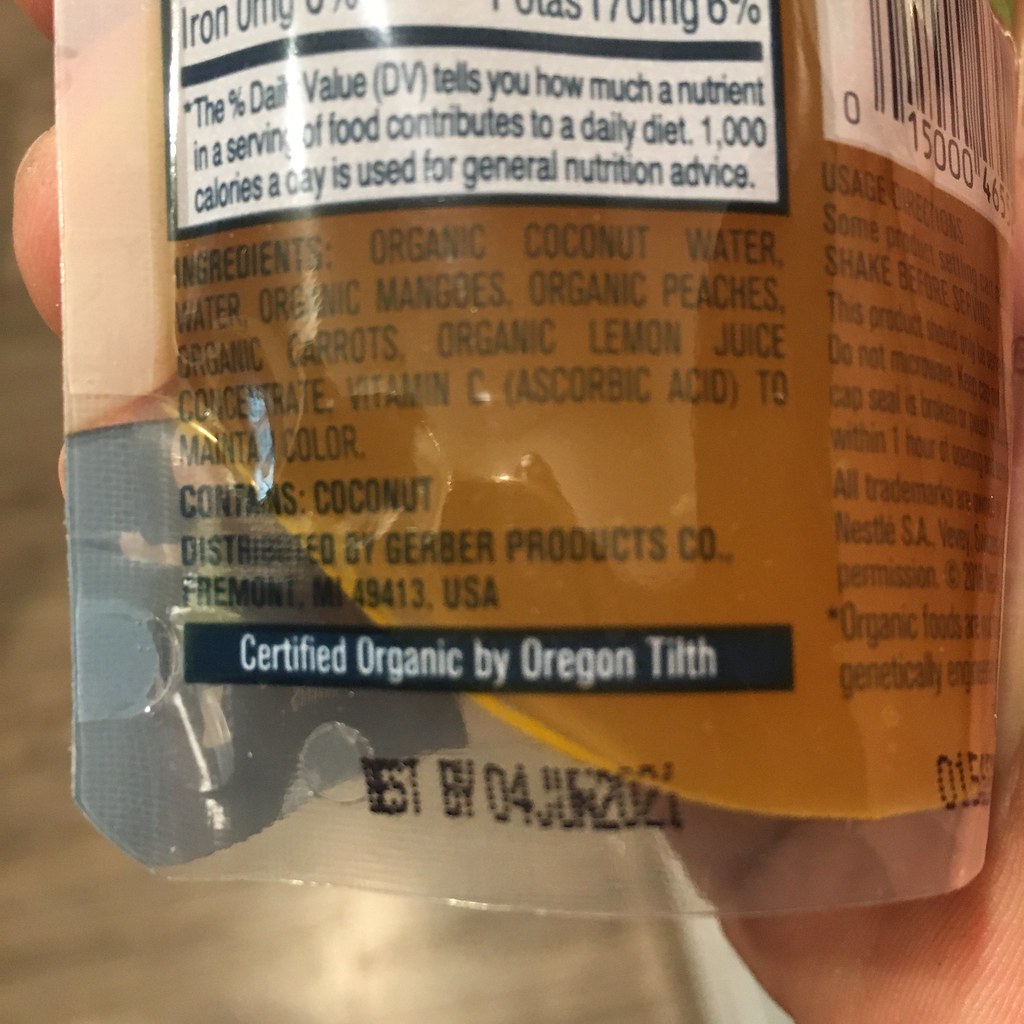This color photograph captures a close-up of a portion of the back label of an organic coconut water container. The container is being held by a person with very pale skin, likely of Caucasian or Asian descent, and only their right hand is visible. The index finger of the person's hand is positioned at the upper left-hand corner of the container, with part of the palm also shown in the frame.

The label on the container details several organic ingredients, including organic coconut water, organic mangoes, organic peaches, organic carrots, and organic lemon juice. Some of the text on the label is partially obscured, though it is clear that the product is certified organic by Oregon Tilth. Additionally, the best-by date is prominently displayed at the bottom of the label, marked as June 4th, 2021. The container appears to be a single-serve package, adding convenience for on-the-go consumption.